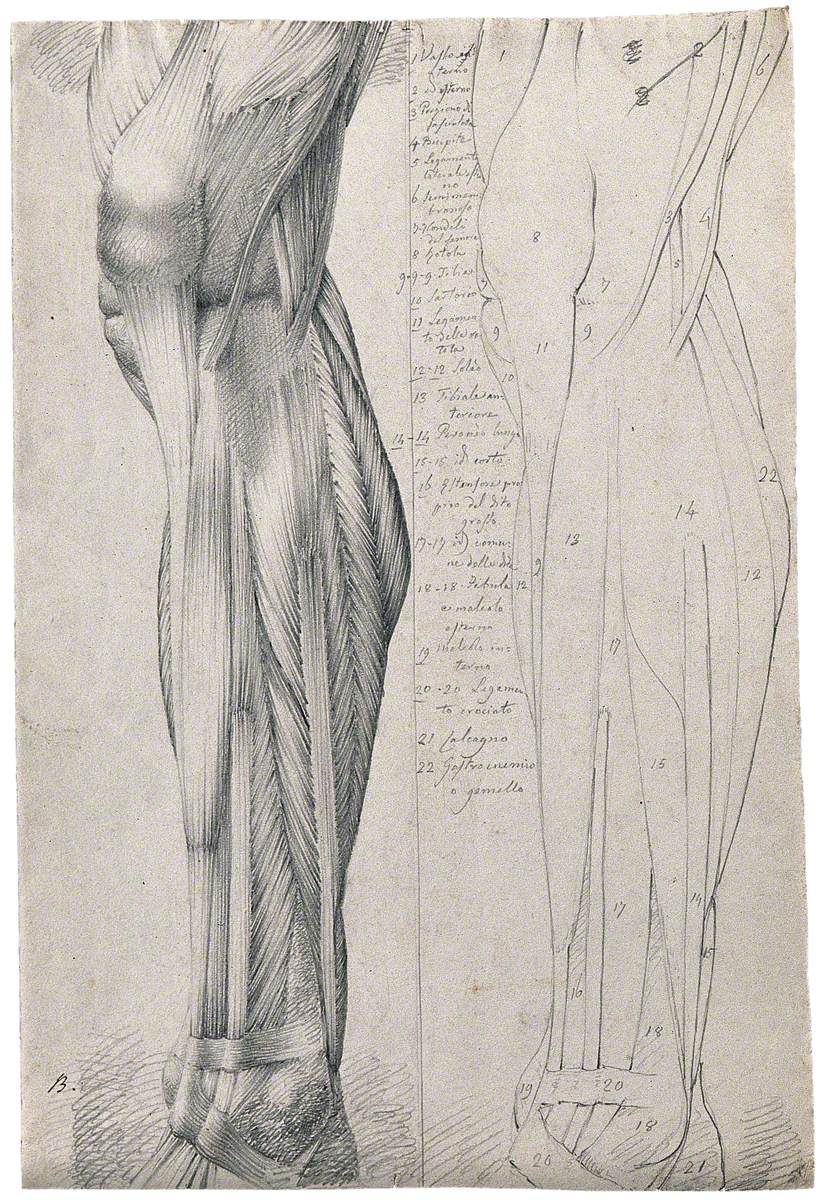The image showcases a detailed, pencil-drawn anatomical diagram of a human leg from the thigh down to the ankle, illustrating the muscular tissues and tendons. The left segment of the image reveals the complex muscle fibers, tendons, and kneecap coverings in an animated manner, while the foot is not visible. The right segment presents a simplified outline of the leg, bordered and labeled with numbers ranging from 1 to 22. Pencil scribbles are evident at the top left and bottom of the off-white paper, suggesting an intricate and meticulous sketching process. The entire diagram is monochromatic, relying on varying shades of black, white, and gray for depth and detail, with a letter "B" marking the bottom left corner. Adjacent to the images are descriptions corresponding to the numerical labels, further elucidating the anatomical features depicted.